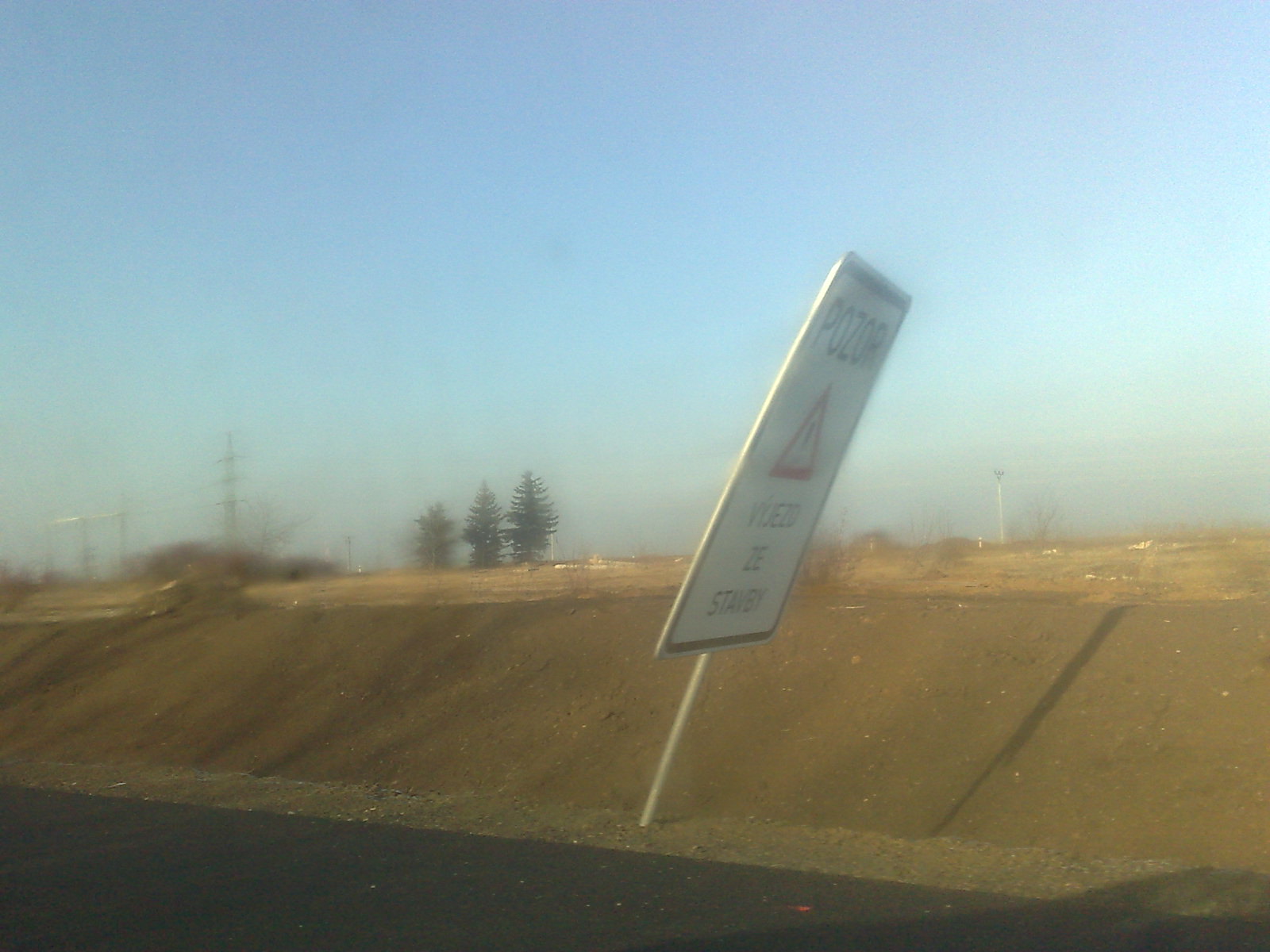A roadside scene featuring a slightly crooked traffic sign mounted on a white pole is captured in this image. The sign is predominantly white with a dark border and displays text in a foreign language, which appears to start with "P-O-Z-O-R." Although the angle of the photograph obscures some details, the prominent feature of the sign is a red triangle in the center with an exclamation mark inside, indicating a warning. Beneath the triangle, there is additional text that is partially legible, potentially reading "D-E" and what might be "standby" at the very bottom.

The sign is situated beside a tarred road or parking lot. Adjacent to the sign, a brown dirt slope ascends to a flat terrain, which is dotted with patches of weeds and small vegetation. In the background, three mature trees stand alongside several telephone or electricity poles to the left. Above, the sky is a serene light to medium blue, void of clouds, suggesting a clear day.